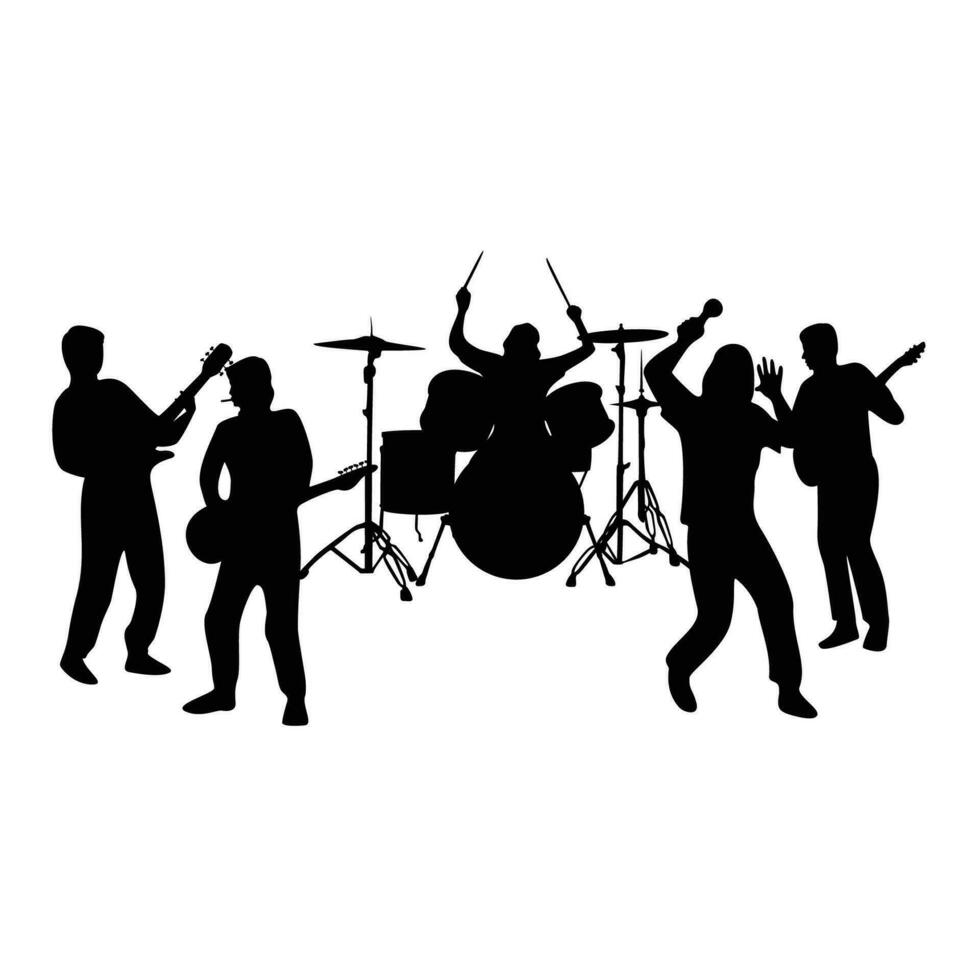The image depicts a striking black and white silhouette of a five-member rock band performing against a stark white background. From left to right, the band is arranged as follows: the first guitarist is leaning slightly backward with his right side facing the viewer, holding his guitar in a classic rock pose. Next to him is another guitarist identifiable by the cigarette in his mouth. Central to the image is an elaborate drum kit featuring a central bass drum, two smaller drums, a large drum to the left, and three cymbals. The drummer is captured mid-action with both drumsticks raised high, hinting at a dynamic performance. To the right of the drum kit stands the vocalist, who holds a microphone in his right hand while his left hand is outstretched dramatically. The final figure on the far right is another guitarist looking back towards the drummer and the rest of the band, perhaps the rhythm guitarist. All these elements combine to form a vivid silhouette representation without any facial or clothing details, emphasizing the energetic postures and the instruments of the musicians, creating a visually compelling image.